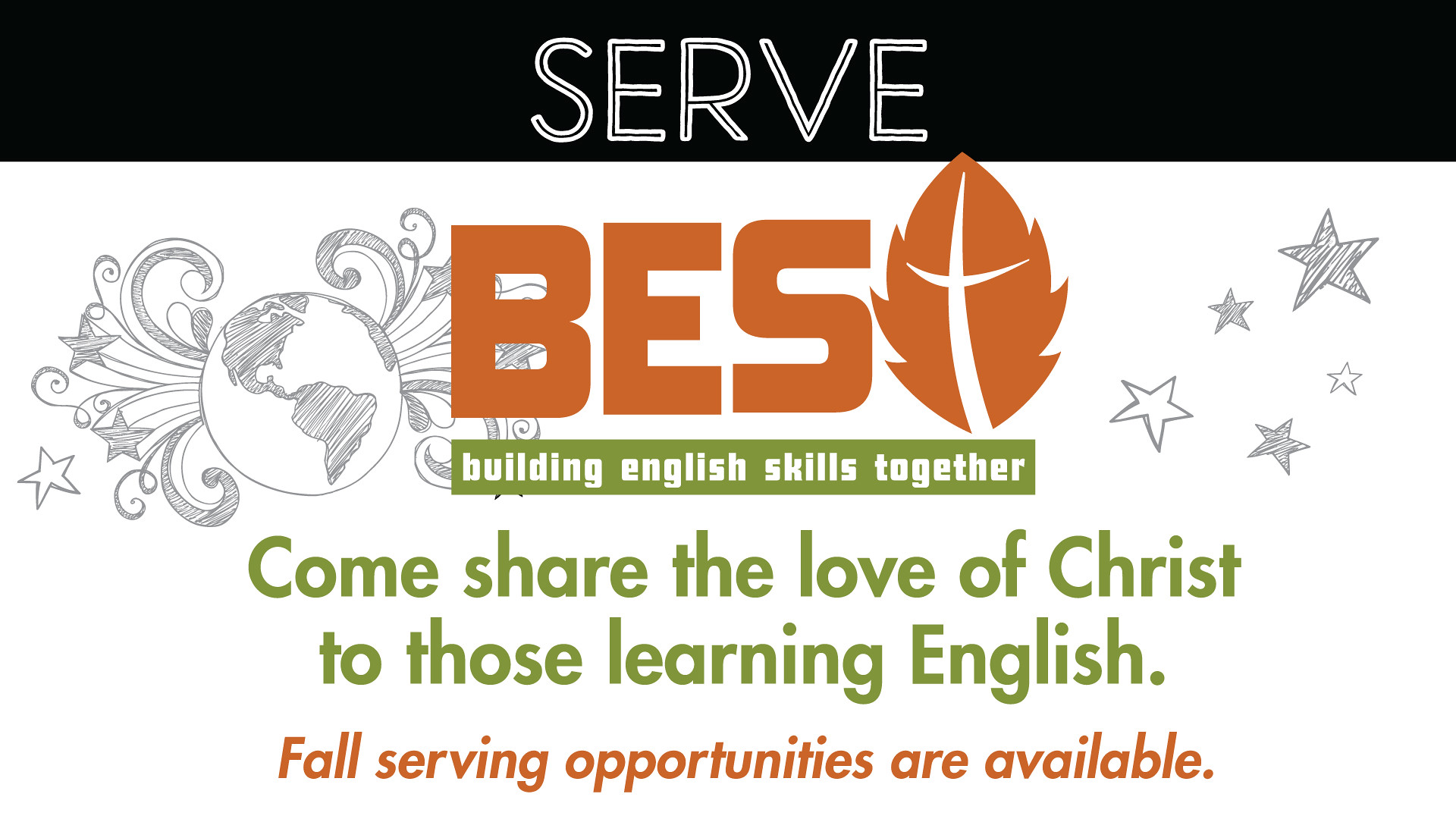This image is an advertisement calling for volunteers to help build English skills while sharing the love of Christ. At the very top, the word "SERVE" is prominently displayed in white block letters on a long black horizontal rectangle. Directly below, "BEST" is written in bold brown capital letters with the T stylized as a cross inside a brown leaf. The phrase "Building English skills together" is presented below in white letters on a green background. Further down, it reads "Come share the love of Christ to those learning English" in green text, followed by "Fall serving opportunities are available" in brown. The background features a hand-drawn image of the earth, complemented by decorative elements and scattered stars, enhancing the visual appeal and emphasizing a global outreach theme.